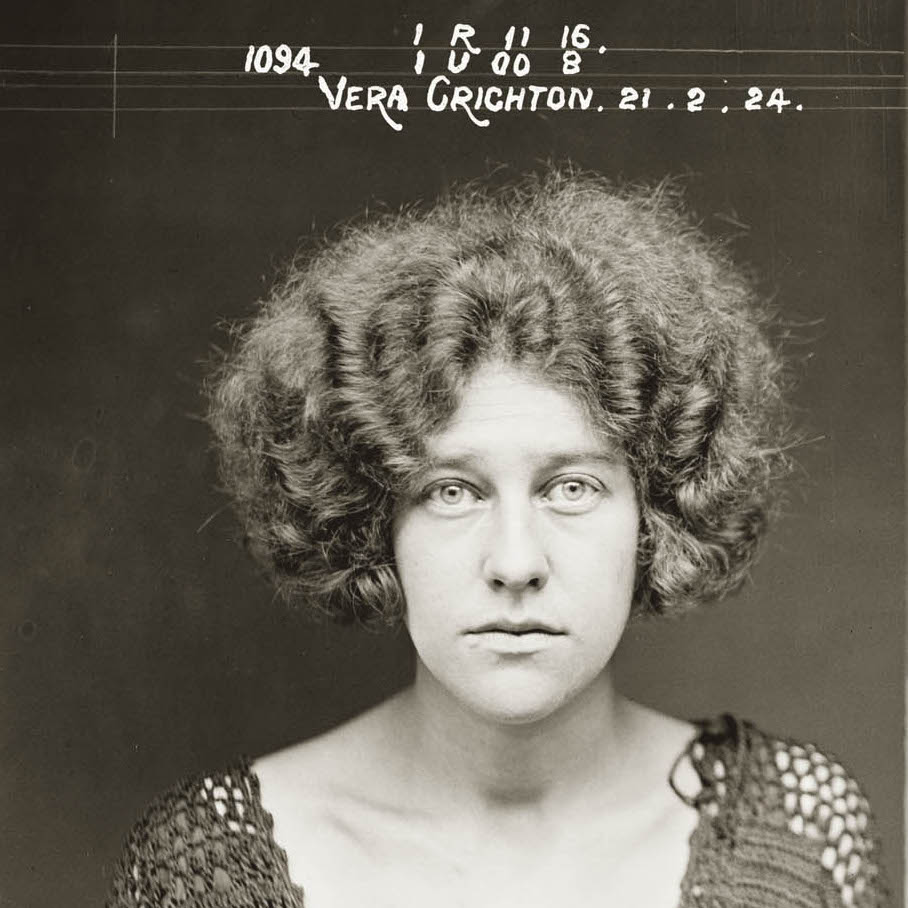This sepia-toned photograph, resembling a black-and-white grayscale image, portrays a young woman in her late twenties named Vera Crichton. She gazes directly into the camera with a serious, almost haunted expression. Vera's face is elongated and oval-shaped, further accentuated by her short, thick, and naturally curly hair, reminiscent of a brillo pad or an afro that frames her head and extends just below her ears.

Vera's piercingly light-colored eyes and lack of makeup highlight her pale complexion. She is dressed in a knit garment, possibly a dress, that features a scalloped neckline and lace details along the shoulders. The garment appears somewhat low-cut, revealing her collarbones and allowing a glimpse of her skin through the open lacework. Notably, the knitwear is coming unraveled, adding a sense of fragility to her appearance.

The background of the photograph is a monochromatic black or dark brown, providing a stark contrast to Vera's pale figure. At the top of the image, there is some text in white, including a series of letters and numbers: "1094, IR 1116, IU 008." It also states "Vera Crichton" and a date that is formatted in the European style: "21.2.24," likely referring to February 21st, 1924. Though the exact context of the photograph remains unclear, it carries an evocative air, resembling a mug shot or an album cover.